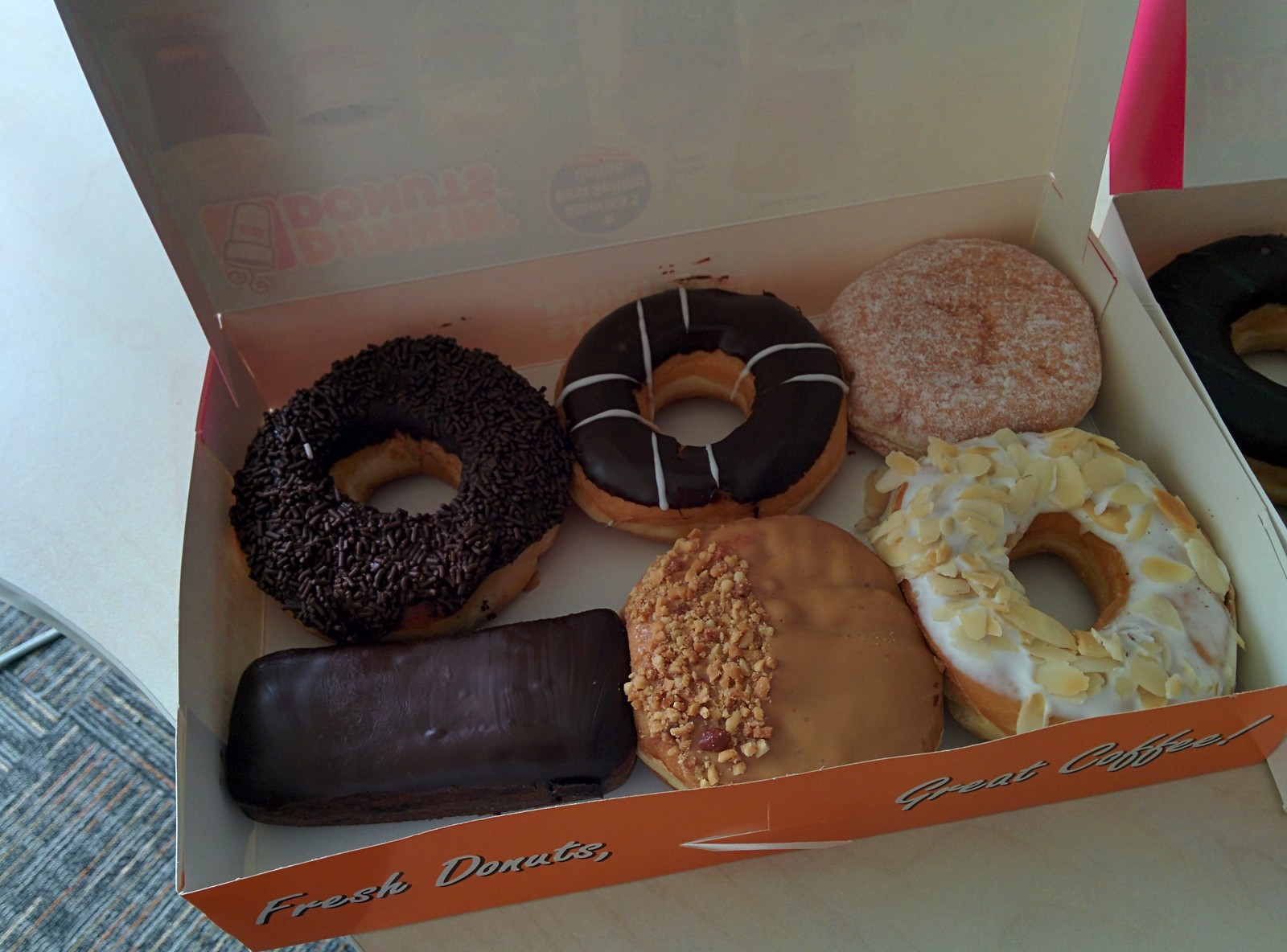The color photograph captures a pair of donut boxes on a table, with the primary focus on an open Dunkin' Donuts box containing half a dozen assorted donuts. The box is predominantly white with an orange edge, displaying the text "Fresh Donuts, Great Coffee!" in white print. The lid of the box is flipped open, and the light allows the Dunkin' Donuts branding to be faintly visible through the top. Inside, the donuts exhibit a diverse assortment: 

1. A large, round donut with chocolate glaze and chocolate sprinkles located at the top left.
2. Next to it, another glazed donut with a chocolate glaze adorned with white icing decorations.
3. The middle donut appears to be jelly-filled, coated in powdered sugar.
4. At the bottom left, there's an eclair-shaped donut fully dipped in chocolate.
5. Adjacent to the eclair-like donut is a jelly-filled donut with a butterscotch or peanut butter glaze, topped with chopped peanuts.
6. Lastly, a round donut with a thick white glaze garnished with slivered almonds lies at the bottom right.

Additionally, a glimpse of another donut box can be seen at the very right edge of the photo, containing only a single chocolate-glazed donut visible from its top corner. The setting appears to be an office or break room, evidenced by the visible commercial-grade carpet in the bottom left corner.